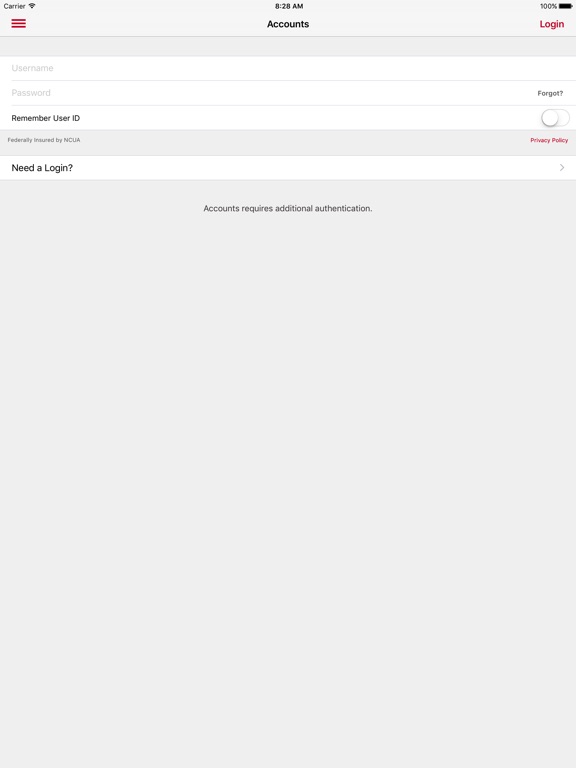In this image, we see a screenshot of a mobile login interface. The background transitions smoothly between gray and white. In the top-left corner, black text reads "Carrier," accompanied by a Wi-Fi icon to its right. Centrally positioned at the top, the time is displayed as 8:28 AM. In the top-right corner, a battery icon indicates a full charge at 100%.

Dominating the center of the screen, "Accounts" is written in bold black text. To its right, in striking red text, is the word "Login." Directly below these headings are input fields labeled "Username" and "Password."

Beneath the password field, a statement reads "Remember User ID," accompanied by a toggle switch on the right. Further down, text indicates "Federally insured by NCUA," positioned next to a link labeled "Privacy Policy."

On a stark white background below these elements, a prompt reads "Need a Login?" with an arrow pointing to the right, directing users to additional login options or help.

At the bottom of the screen, encompassed in a large gray box, a centered message in black text informs the user that "Accounts requires additional authentication."

This detailed breakdown offers a comprehensive understanding of the visual and textual elements present in the screenshot.